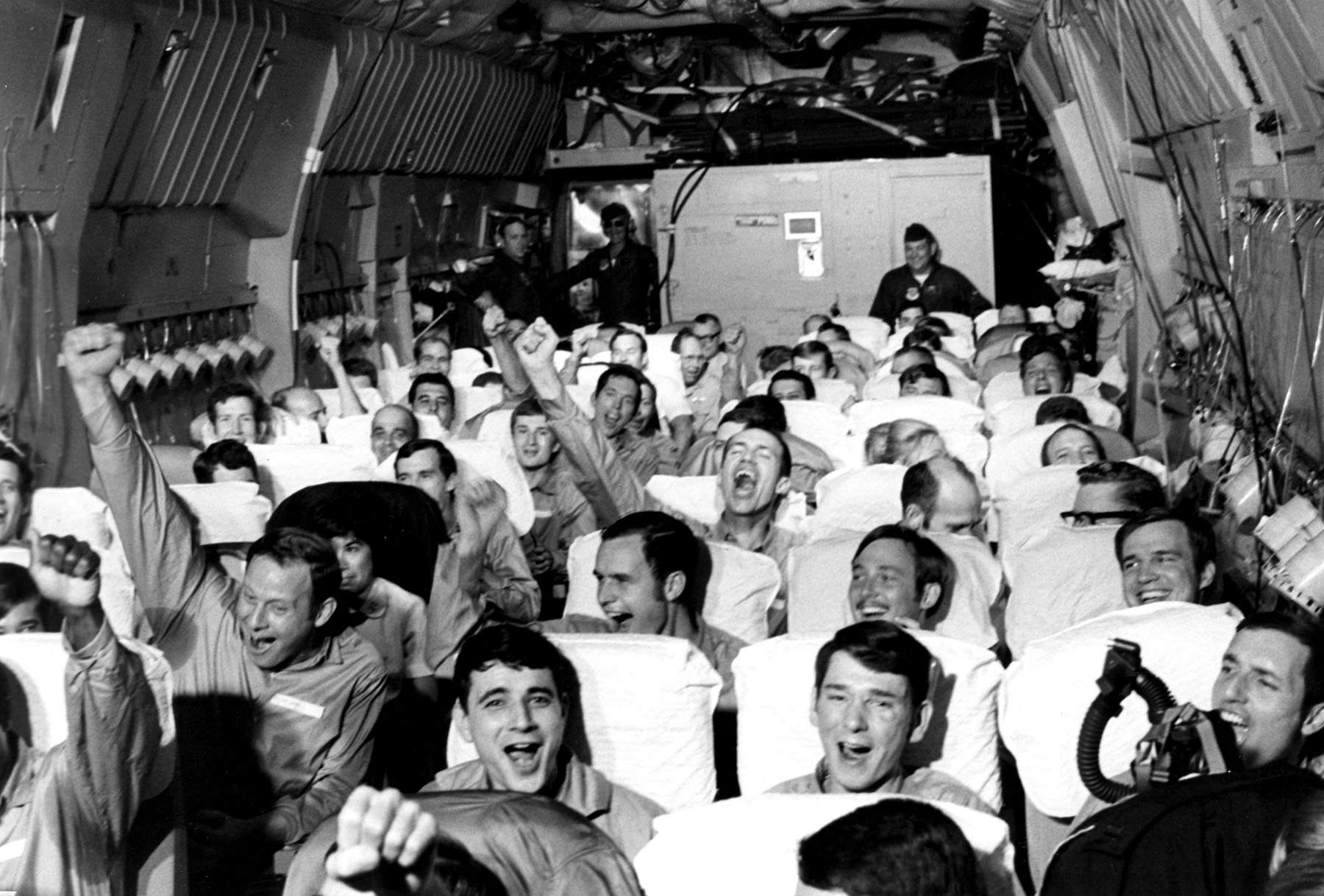This black and white photograph depicts the inside of the back end of a military airplane. The image showcases a jubilant scene with several rows of seats, each topped with white pillows, occupied by men wearing long-sleeved gray shirts. Some of these men have their arms extended upward and their mouths open, appearing to cheer and celebrate, possibly indicating they've received good news or are heading home after a mission. The plane’s interior has rounded, dome-shaped walls adorned with wires, equipment, and oxygen masks hanging from tubes. In the background stands a large, metallic box, taller than the men, with a man in an army uniform seated in front of it, grinning as he presumably speaks through a microphone, further suggesting the aircraft's military use. The photograph, seemingly from the 70s or 80s based on the hairstyles of the men, conveys a poignant moment of joy and relief among these servicemen.